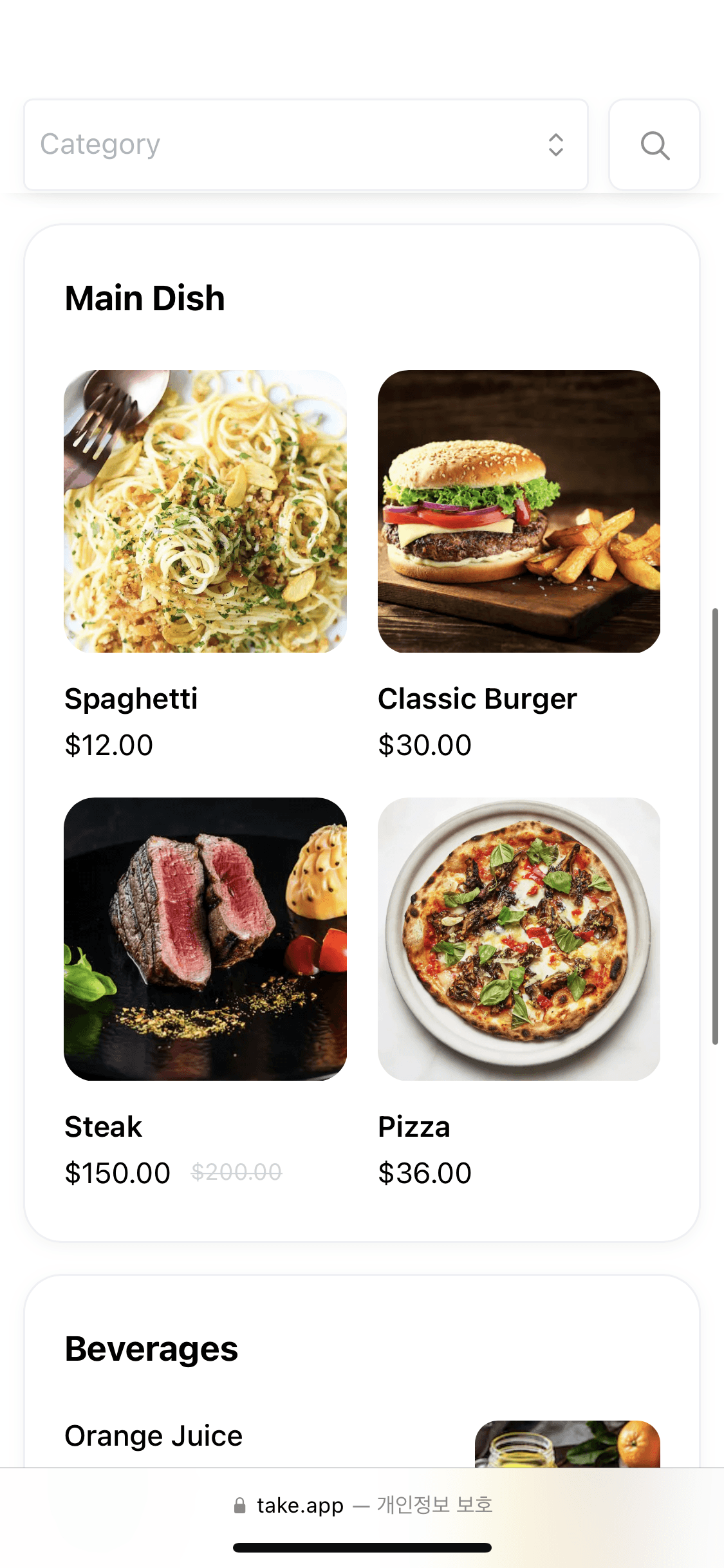This is a detailed screenshot of what appears to be an online restaurant menu, possibly from a food delivery app similar to Uber Eats, though no specific logo is present to confirm the platform. At the top of the screenshot, there's a search bar labeled "Category," which currently has no category selected. To the right of the search bar, there's a magnifying glass icon, presumably for initiating a search after selecting a category.

Below this search section, the menu lists the "Main Dish" category, showcasing four distinct food items, each displayed within its own box:
- **Top Left**: Spaghetti priced at $12.
- **Top Right**: Classic Burger priced at $30, accompanied by a side of fries as depicted in the image.
- **Bottom Left**: Steak priced at $150, suggesting a high-quality or large portion.
- **Bottom Right**: Pizza priced at $36.

At the very bottom of the screenshot, there is a section labeled "Beverages," with only "Orange Juice" visible, implying that there are additional beverage options not shown in the current view.